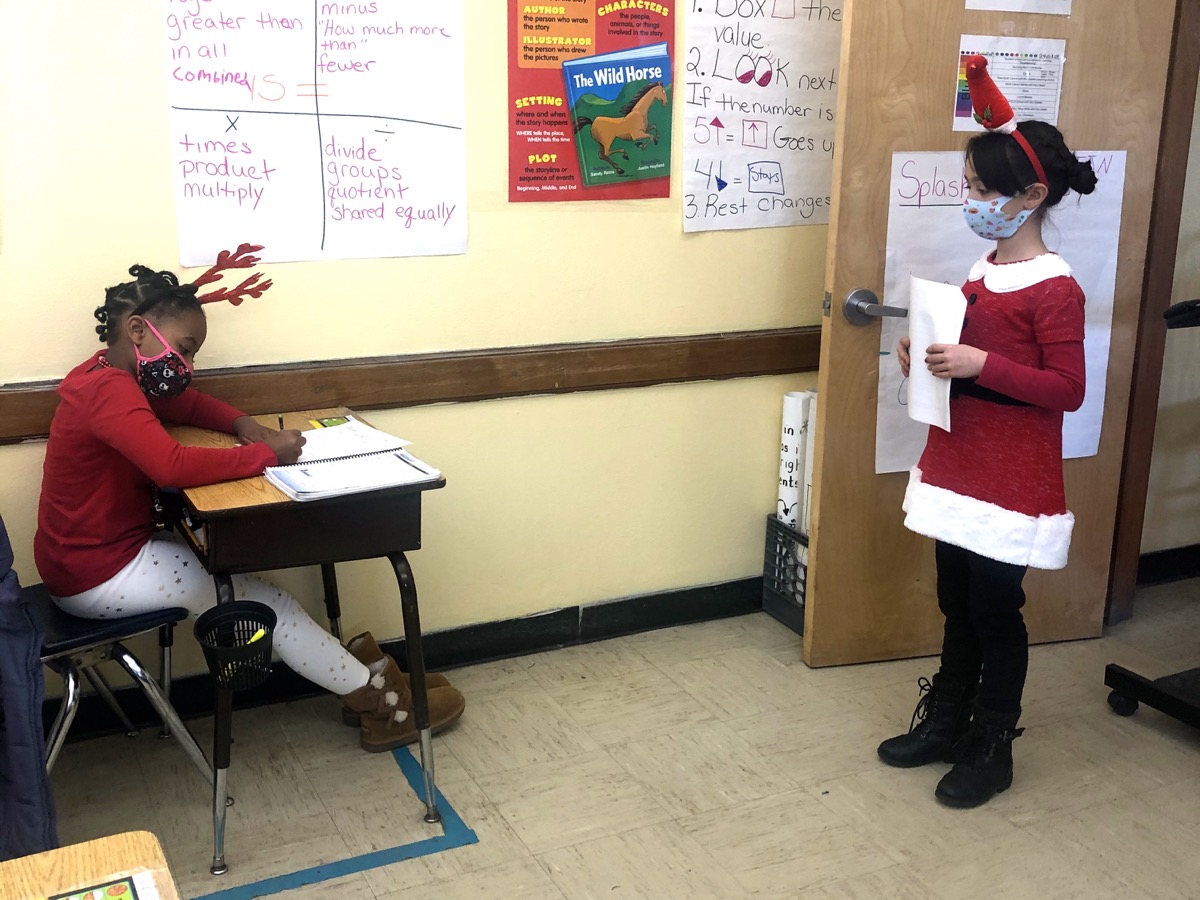In this detailed and festive classroom scene, around the holiday season, two young students are immersed in their activities. On the left side of the room, a young African American girl is diligently working on her homework at a desk outlined by painter's tape to maintain its position. She is wearing brown boots, white pants, a red shirt, and a headband with reindeer antlers. Her face is protected by a pink and black mask. 

On the right side, a young Caucasian girl with black hair stands nearby, holding a piece of paper. She is dressed in a Mrs. Claus-like costume, complete with a red coat trimmed in white, black pants, black boots, and a red long-sleeve shirt underneath. On her head, she sports a headband that features an elf hat and wears a blue mask over her face. 

The classroom's back wall is decorated with posters, including math-related terms such as "greater than, product, multiply, divide, quotient, shared equally," alongside a reading challenge poster featuring a book titled "The Wild Horse." The classroom setting suggests an environment celebrating the holiday spirit, potentially amidst pandemic precautions, with desks maintained at a distance to ensure safety.